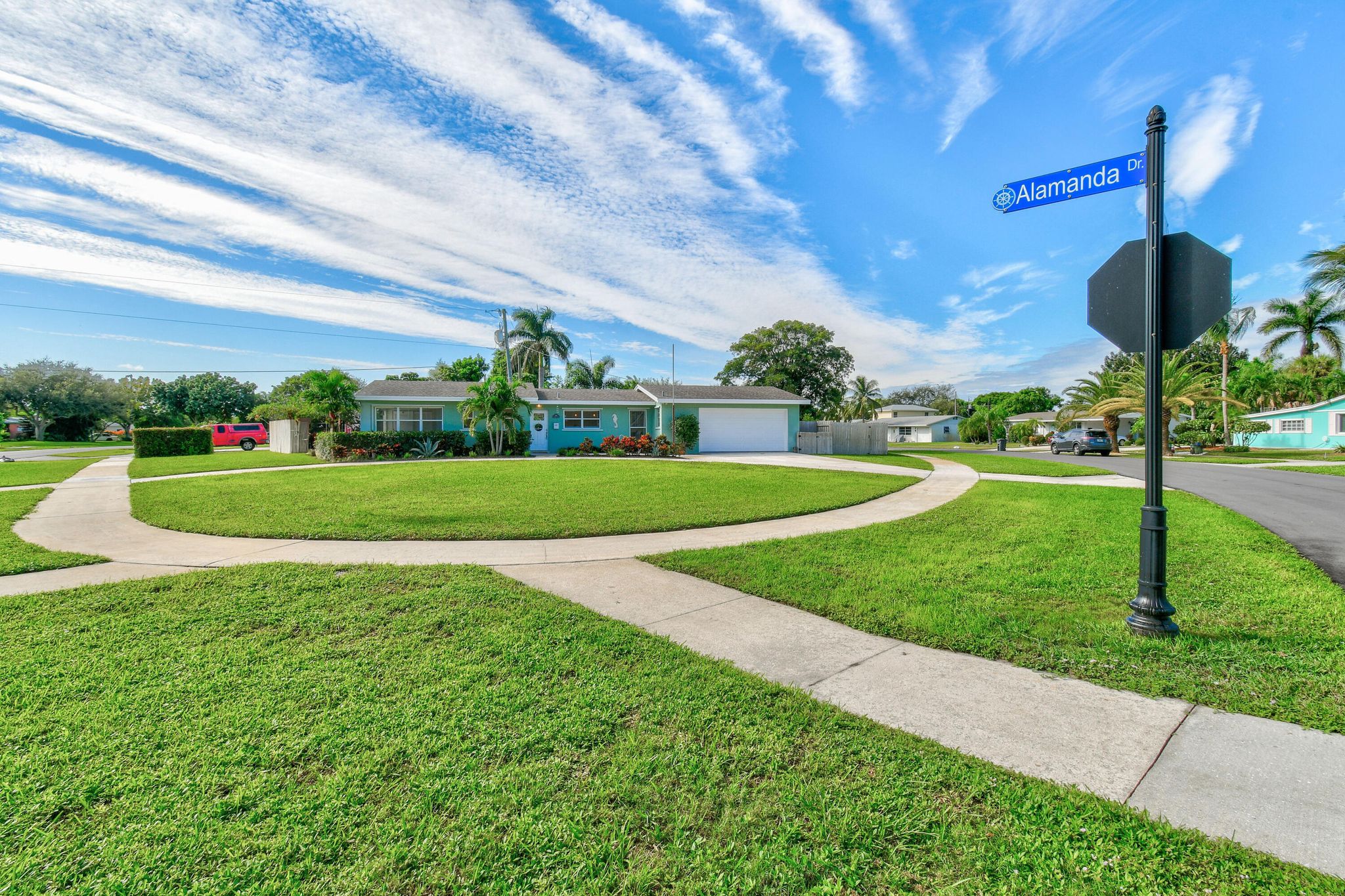The photograph captures a picturesque suburban neighborhood under a bright blue sky adorned with long streaks of clouds. Central to the image is a charming light blue, single-story house with a gray roof, a white garage door, white window frames, and a white entry door. Attached to this house is a neat driveway that leads to the garage, and this is flanked by green grass and meticulously maintained palm trees and bushes. In front of the house, on the grass towards the street, stands a black metal signpost featuring a blue road sign reading "Alamanda Drive," indicating the name of the street. The front yard also showcases a network of intersecting sidewalks, with one prominently curving in an oval shape.

Beyond the primary house, the scene expands to include other homes, adding depth to the neighborhood setting. To the right, another light blue house is partially visible, also adorned with white window frames. Meanwhile, a red SUV is parked in the driveway of the main house, and a blue SUV is seen driving down the black concrete road that separates the houses. Off in the distance, on the right-hand side of the image, there's a small white house with a gray roof nestled among more palm trees, contributing to the lush, tropical ambiance of the neighborhood. This detailed and vibrant image encapsulates a serene and orderly suburban scene.